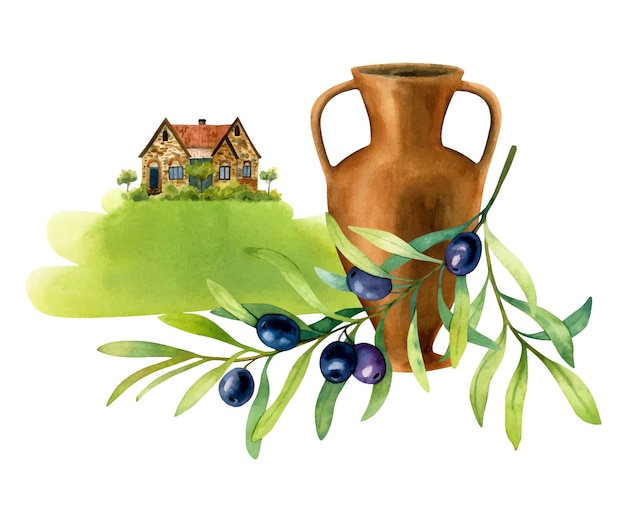The image is a detailed rendering showcasing three main elements. Dominating the center is an almost copper-colored jug, resembling an ancient Greek or Roman water vase, featuring two handles on either side. In the foreground lies a branch adorned with six purple grapes and long, narrow green leaves. In the background, a house is depicted, characterized by a stone exterior and a large green lawn that appears to be on a hill. The house has a door on the left, three triangular roofs facing forward, one triangular roof at a 90-degree angle running the length of the house, three windows, and is surrounded by three trees. The overall scene blends historical elements with a serene pastoral backdrop.